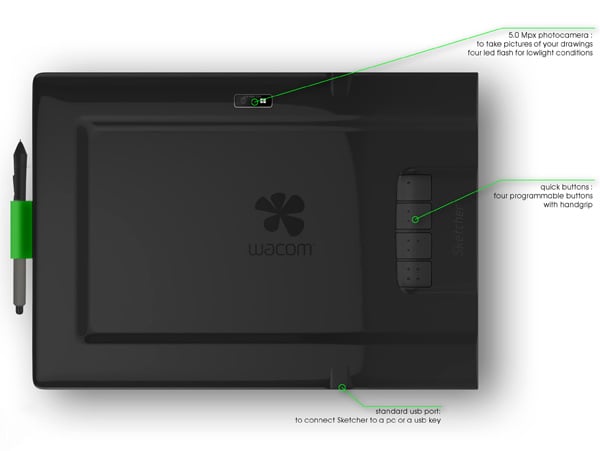This image features a detailed infographic of a Wacom digitizer. The unit, predominantly black with a silver accent, prominently displays the Wacom logo at its center with accompanying informative text. Towards the top of the graphic, a designated rectangular section highlights the device's built-in 5-megapixel photo camera, designed to capture images of your drawings. This camera is equipped with a 4 LED flash to enhance picture quality in low light conditions. 

To the right side of the digitizer, four black quick buttons are identified. These buttons are programmable, offering customizable functionality, and are ergonomically designed with a hand grip for ease of use. Below these buttons, the graphic points out a standard USB port, essential for connecting the digitizer to a PC or a USB key for streamlined data transfer. 

On the left side, a green slot securely holds a stylus that features a two-tone color scheme of black and silver. The infographic uses black callouts to label each component, while green lines effectively connect these callouts to their respective parts on the digitizer, enhancing the clarity and visual guidance of the information presented.